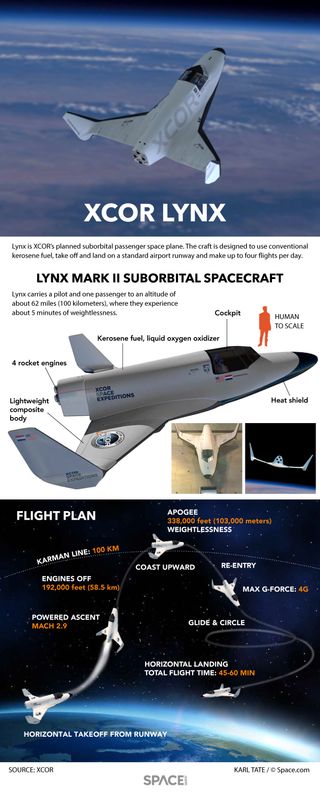The image provides a detailed infographic of the X-Core Lynx suborbital spacecraft. The first of the three panels illustrates the Lynx Mark I in orbit, soaring above Earth's atmosphere, highlighting its function as a suborbital spaceplane. The spacecraft, predominantly white with black and red accents, features a rectangular body with a curved front and four propulsion units at the back. Its large wings extend from the rear, flaring upwards. The second panel offers a comprehensive breakdown of the Lynx Mark II, presenting a side view with a human figure in orange for scale. This section labels various parts of the spacecraft, although the text is not entirely legible. The Lynx Mark II is all white with black trim and a prominent black tip, equipped with a sizable front window. The final panel demonstrates the flight plan of the spacecraft. It showcases how the Lynx launches from Earth, ascends into space, and then glides back down, following a spiraling trajectory. Overall, the infographic emphasizes the spacecraft's design and function, aiming to provide brief space trips for passengers to experience Earth's view from above before safely returning.